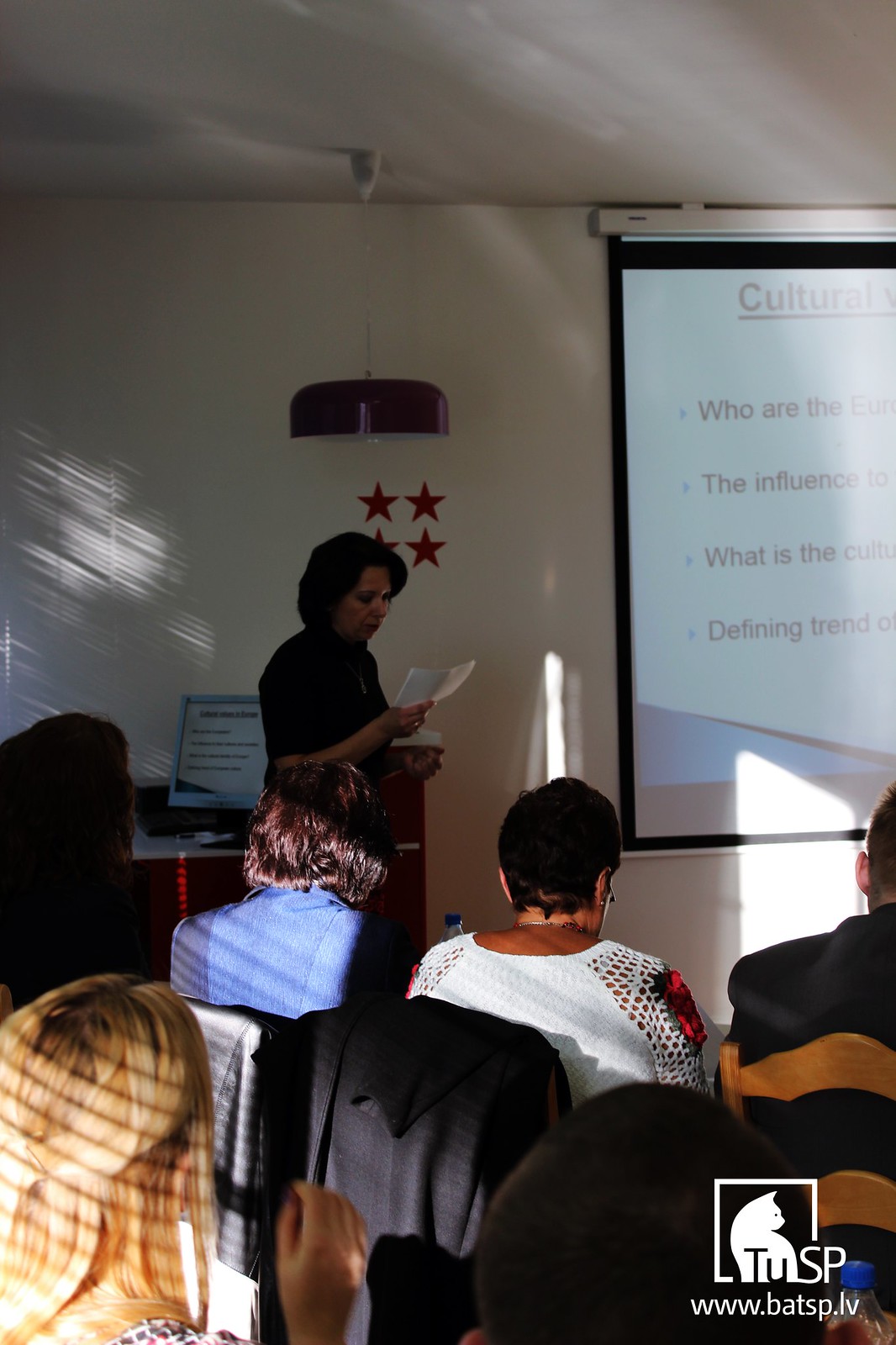The image depicts a classroom setting with a teacher presenting at the front while students sit and listen. In the foreground, five students are seated in two rows, their heads turned towards the teacher, making it difficult to discern their genders. Most students appear to have short hair. A blonde student in the bottom left corner is distinguishable, with her hand up next to her, while another student with dark brown hair sits nearby. 

At the front of the room, a brunette woman with short hair, wearing a dark short-sleeve blouse, stands and reads from a piece of paper held in her right hand. To her left, there is a computer on a table, which mirrors what’s shown on the projector screen to her right. The screen displays text, with visible words such as "cultural" and fragmented phrases like "who are the influence" and "defining trend."

In the background, the wall is white, and a set of four red stars arranged in a square is noticeable just above the teacher, along with a dark-colored ceiling light. Sunlight floods through windows, casting glares on the backs of some students and reflecting on the wall. At the bottom right of the image, a logo featuring a cat and the letters T-U-S-P appears next to the website "www.batsp.lv."